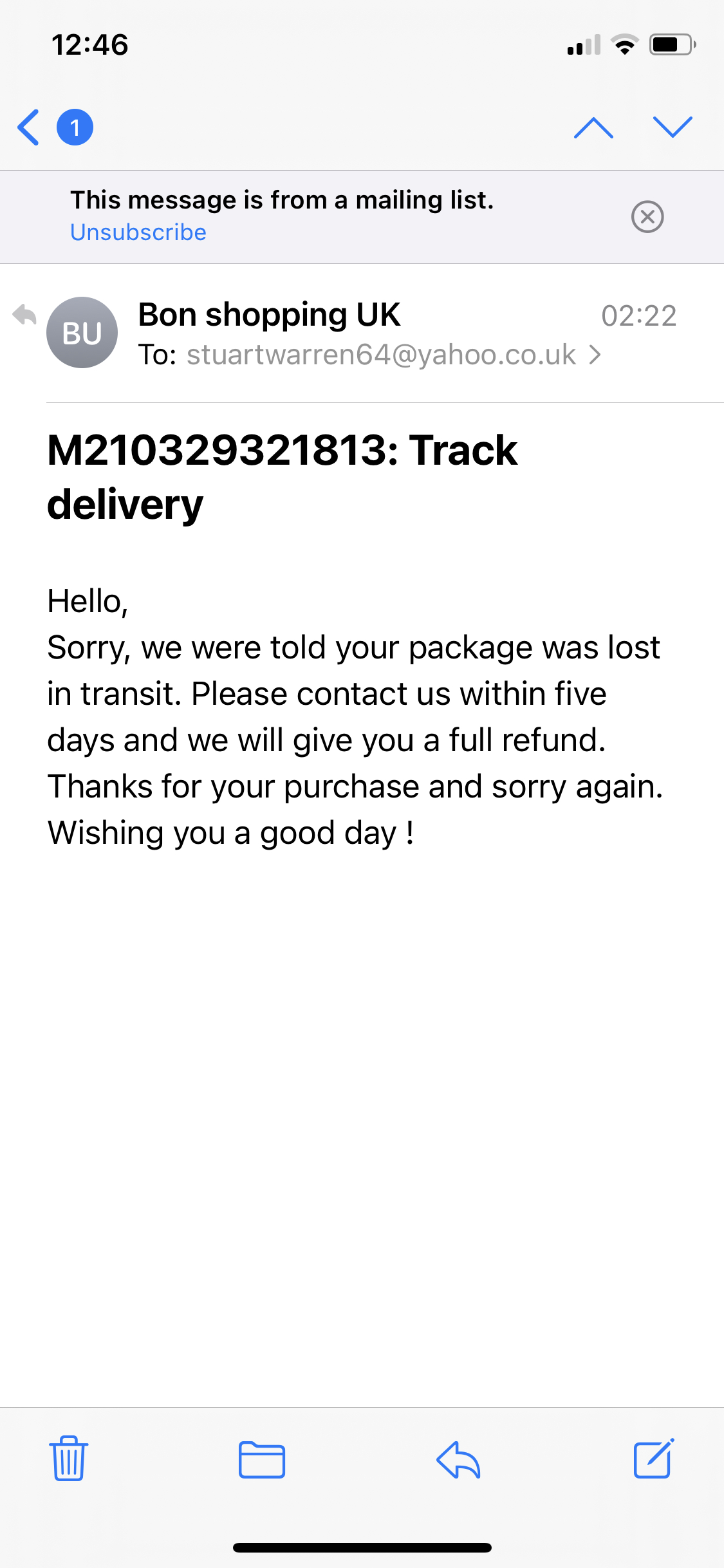**Detailed Descriptive Caption:**

The image is a screenshot of an email displayed on a device. The device shows the time as 12:46 at the top left corner, and the battery indicator at the top right corner indicates approximately 70-75% charge. Directly below the battery indicator is a notification stating, "This message is from a mailing list."

The sender of the email is identified as "Ron or bond shipping UK." The email is addressed to "StuartWarren64@yahoo.co.uk" and was sent at 2:22 a.m. The subject line of the email reads: "M2 1 0 3 2 9 3 2 1 8 1 3: Track Delivery."

The body of the email begins with a greeting: "Hello". It then explains that the recipient's package was reportedly lost in transit. The message requests that the recipient contact the company within five days to receive a full refund. The email concludes with an apology and well-wishes: "Thanks for your purchase and sorry again. Wishing you a good day."

Additionally, at the bottom of the email, there is a hyperlink in light blue text that allows the recipient to unsubscribe from the mailing list.